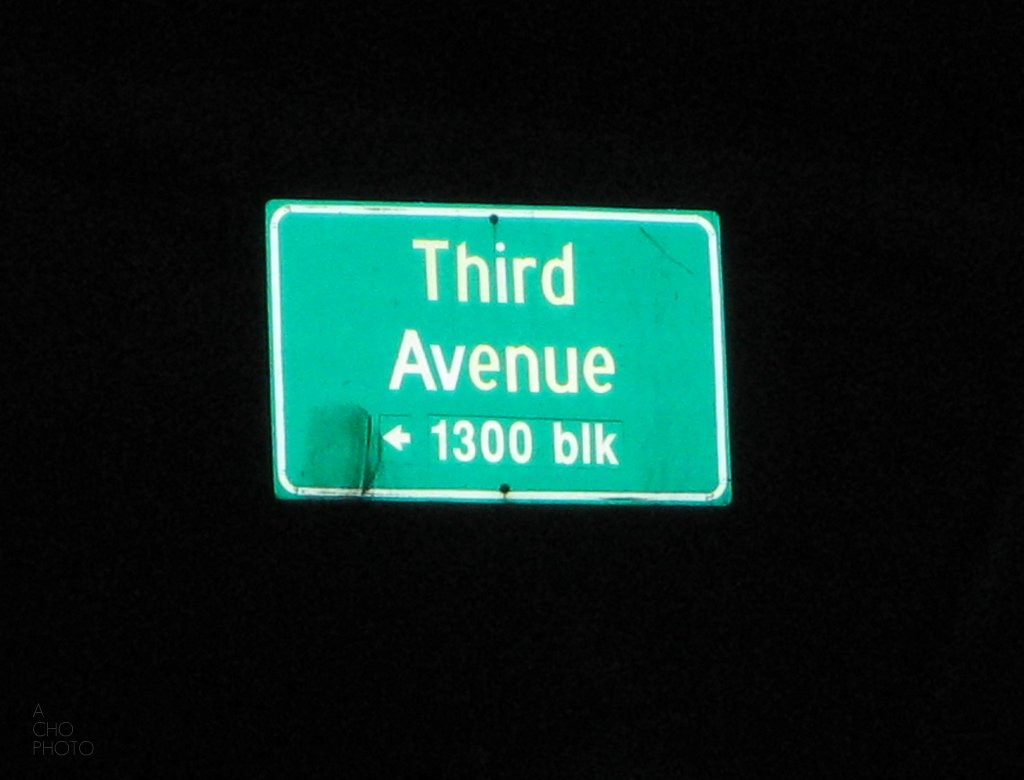In this nighttime outdoor photograph, the plain black background emphasizes the solitary, illuminated object at its center: an aged green and white road sign. The sign's prominent white border frames its content—a stark contrast to the dark surroundings. In crisp white lettering, the sign reads "3rd Avenue." Directly beneath this text, a left-pointing arrow provides directional guidance, and the additional designation "1300 BLK" identifies the block number. The sign's weathered appearance, marked by discoloration, imperfections, and various black lines that resemble scratches, hints at its long service. Moreover, a smeared black patch further testifies to its age and exposure to the elements. Despite its worn condition, the sign glows brightly, drawing the viewer's eye and standing out as the lone illuminated feature in the composition.